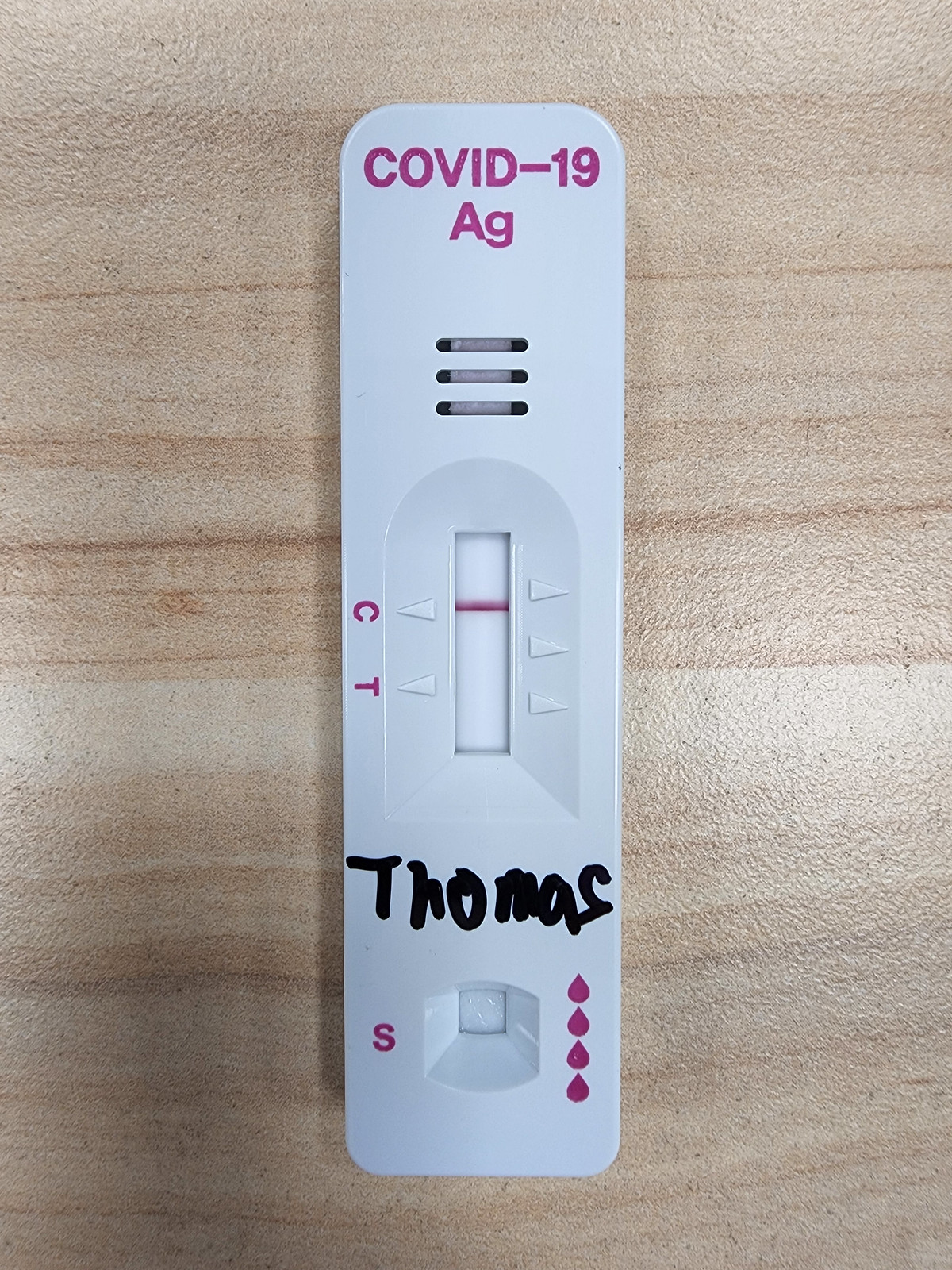This image captures a detailed view of a white COVID-19 test kit, placed on a brown table. On the top of the test kit, "COVID-19" is prominently written in red or pink. The test kit features three sequential openings, aligned vertically. A U-shaped opening with a flat bottom is present on the main body of the kit. Adjacent to the U-shaped opening, there are three triangular designs pointing to the right and two pointing to the left.

Below these designs, "CT" is inscribed horizontally, accompanied by a red line between the first set of triangles. Further down, the name "Thomas" is written in black ink. At the bottom of the test kit, the letter "S" is visible on the left side. Additionally, there is a small screen with square corners nearby, displaying what appears to be four pink droplets.